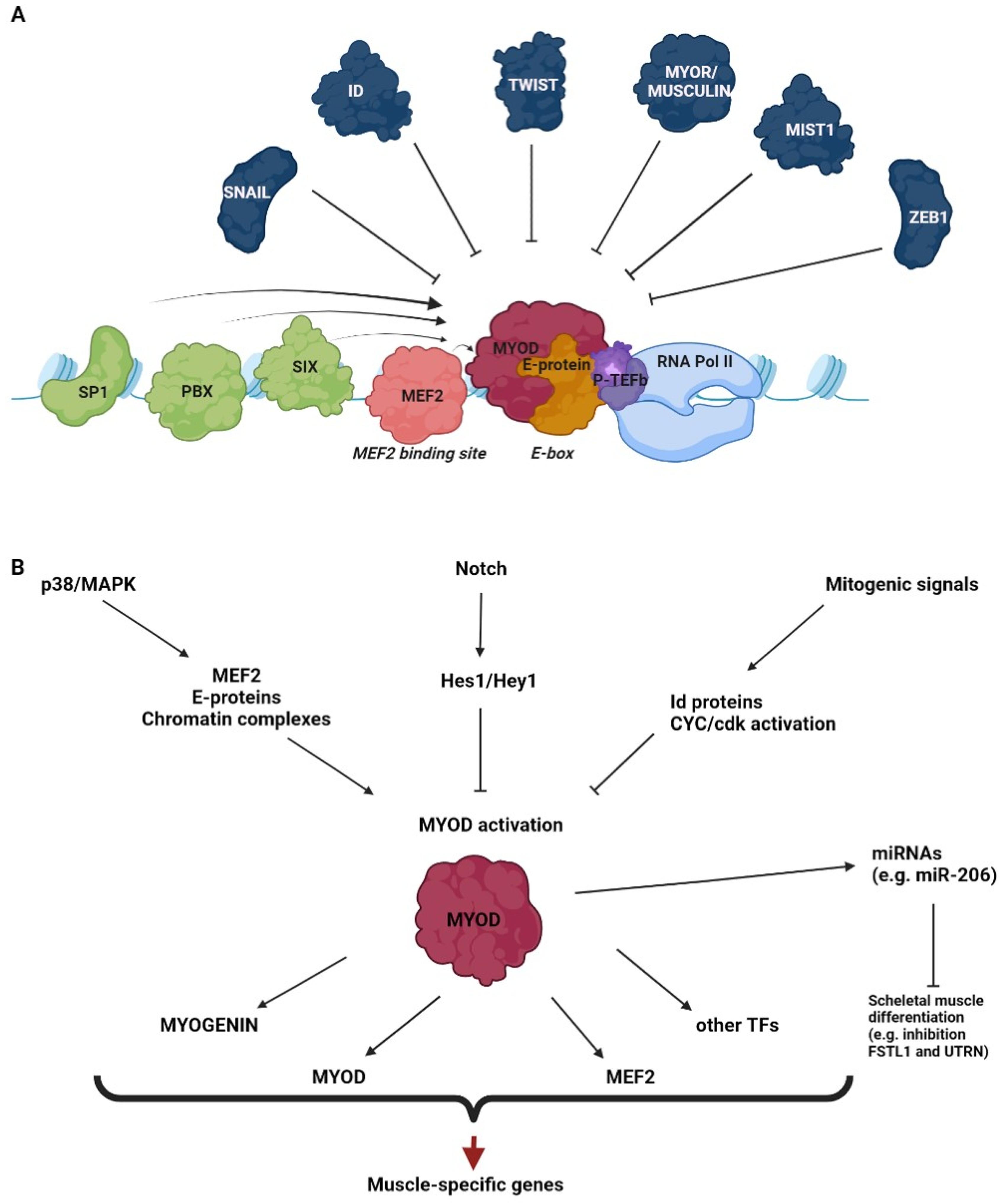The image is a detailed, color-coded flow chart from a scientific paper or textbook, depicting the effects of various proteins on musculature tissues, culminating in muscle-specific gene expression. The chart is divided into two main sections, labeled A and B. Section A resembles a traditional mind map with MYOD at the center, surrounded by arrows indicating the activation of MYOD and interactions with other factors such as transcription factors (TFs), MPOD, myogen, chromatin complexes, and ID proteins. This section features cloud-like shapes in colors like navy blue, green, pink, dark pink, orange, purple, and light blue, each corresponding to different proteins and their roles. Text within these shapes includes SNAIL, ID, TWIST, MAO, MIST1, SERP1, SP1, PBX, MEF2, and RNA Pol II. The flow chart illustrates connections between these proteins and processes, such as chromatin remodeling, CDK activation, and mRNA translations, ultimately leading to muscle-specific genes. Section B, positioned below, is similarly organized and further details this complex interplay, reinforcing the connections to muscle-specific gene expression. The coherent visualization through arrows and color-coding allows for easy identification of components and their biological significance.